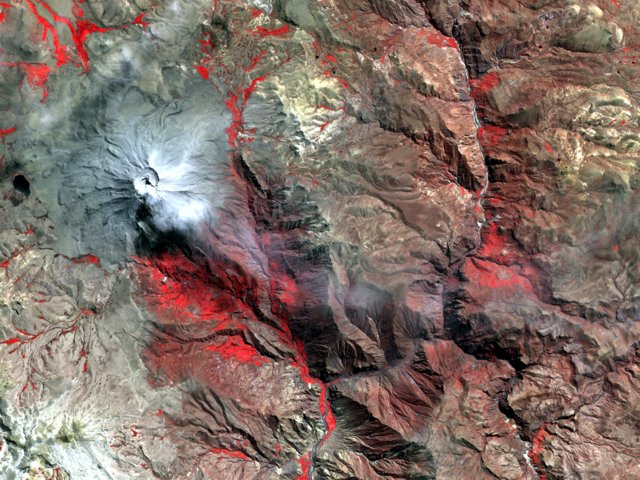The image is a square, borderless, multicolored photograph characterized by a rugged, rocky terrain. Dominated by shades of whitish, reddish, and grayish colors, the photograph lacks any people, text, or animals. The scene prominently features a volcano-like structure near the center-left, identified by an oval indentation at the top and surrounded by lighter, white-colored mineral deposits which may represent the highest elevation in the image. Scattered vivid red areas, particularly around the top left and center, appear to be lower-lying valleys amidst the predominant dark gray, rocky, and jagged landscape. The perspective seems to be an aerial view, adding a layer of abstraction to the already color-graded and texturally varied terrain, making identification challenging.